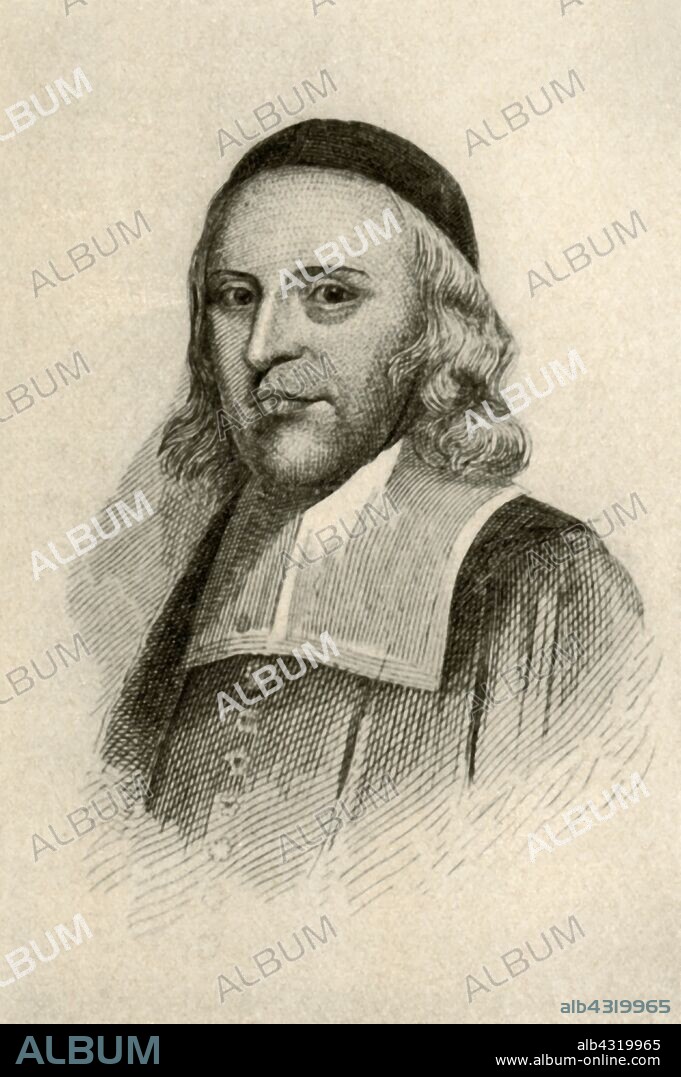This image is a detailed, hand-drawn black and white sketch of John Leverett, the former governor of Massachusetts during the colonial era in the 1600s. Leverett is depicted from the chest up with distinctive long hair falling to his shoulders and wearing a colonial-era black outfit featuring a white collar. He completes his attire with a black hat. The background of the sketch is a light beige color, which has aged to a yellowed tone over time. Scattered across the drawing are persistent watermarks alternating in white and gray that read "ALBUM" in capital letters. At the bottom of the image, there is a black rectangular strip where more text is present. This text includes the word "ALBUM" again in a different typeface, a reference number "ALB4319965" in white, and a URL, "www.albumonline.com," also in white. The man’s eyes are noticeably wide open, lending him a very alert expression.